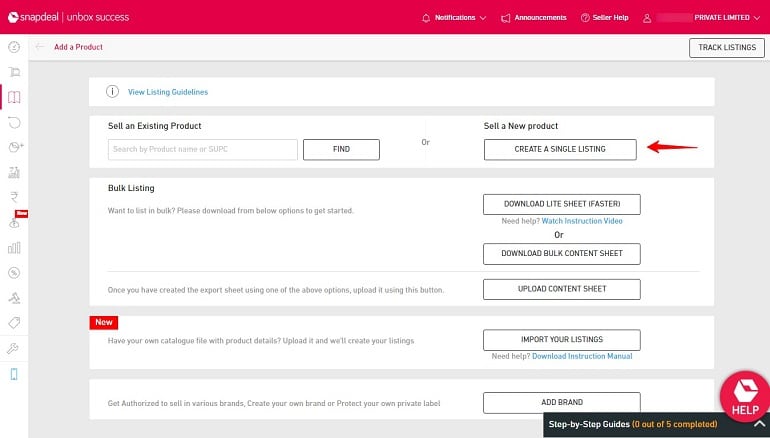The image depicts the product page of an item, predominantly featuring a pink color scheme. In the bottom-right corner, there is a help setting icon available for assistance. Along the bottom of the page, a step-by-step guide indicates "0 out of 5 complete," suggesting a process that needs to be followed. 

Several interactive options are spread across the page, with the first option highlighted by an arrow, indicating the initial step the user should take. Information is dispersed throughout, accessible via clickable sections on both the left side and center of the page. Each clickable item can expand to reveal more details.

At the top of the page, an arrow directs users on where to begin, emphasizing the starting point. Additionally, a purple arrow is visible, pointing to the left, further guiding navigation. This comprehensive layout ensures users can easily find the necessary information and follow the process step-by-step.